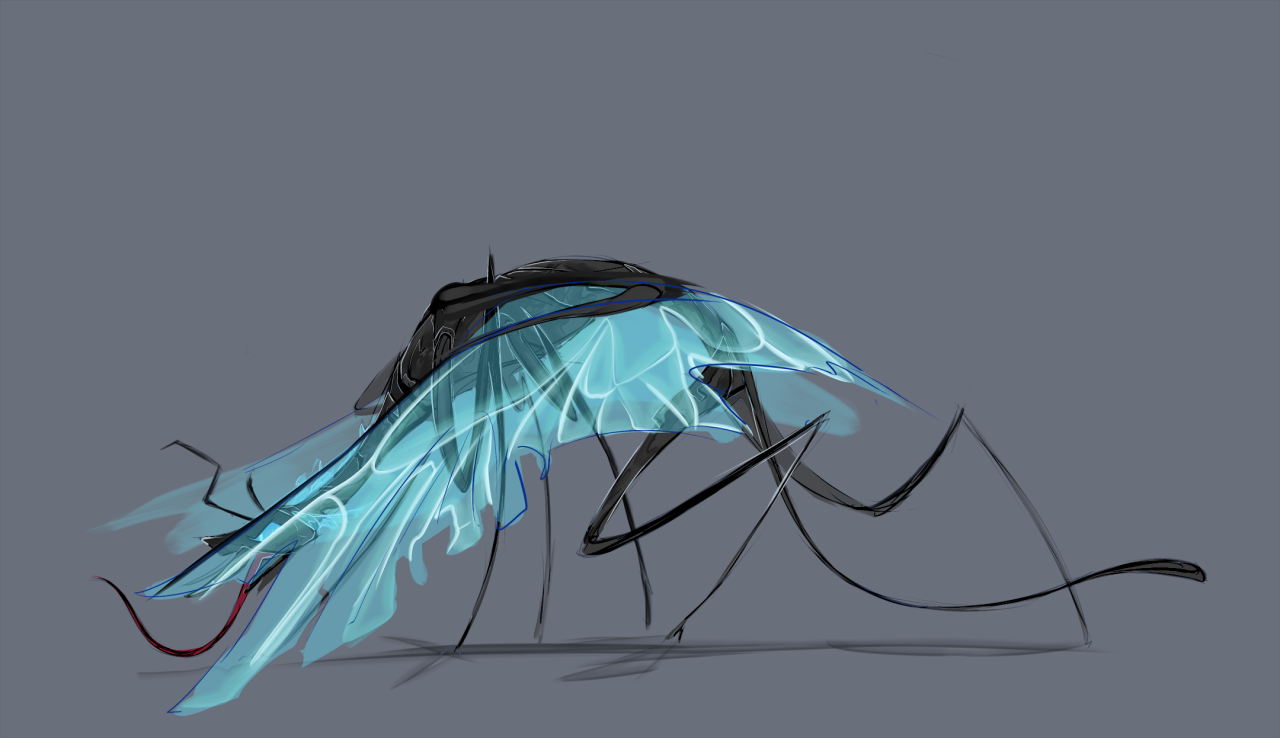The image depicts a digital painting or computer-generated artwork featuring what appears to be a stylized, insect-like creature set against a dark gray background. Central to the composition is the creature, which has a distinct, detailed structure reminiscent of a mosquito. The creature’s body is predominantly dark brown with a head that slopes downward toward the left side of the image. From the head extends a long, slender, red tongue, and its transparent, light blue wings are positioned in a forward-sloping manner, partially revealing sections of its body and face beneath them.

The creature's legs are black, spindly, and double-jointed, forming distinctive U or V shapes that extend toward the ground, suggesting at least six legs. Additional black lines protrude from the creature’s sides, zigzagging in various directions, and a reddish line toward the back gives the appearance of a tail. Despite its complex, articulated limbs and appendages, the entire structure appears balanced and capable of standing upright if it were a physical model. The overall impression conjures an eerie yet fascinating artistic representation that blends elements of realism and abstraction, focusing solely on the creature with no other elements in the scene.